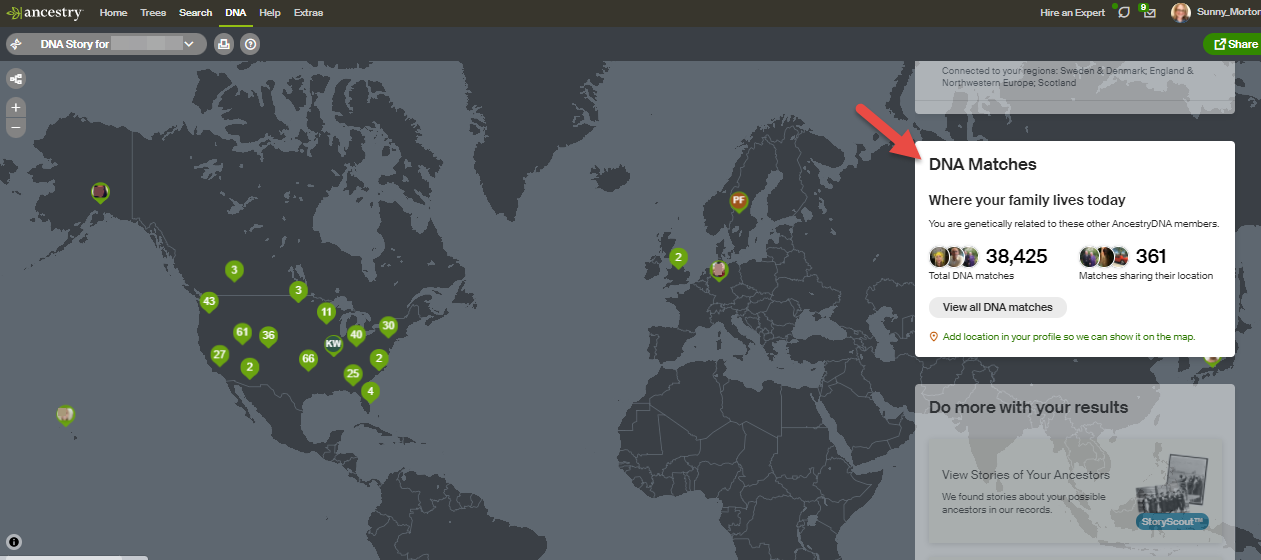**Detailed Description of Ancestry Website Screenshot:**

The screenshot captures the interface of the Ancestry website. Dominating the upper border is a green leaf logo, followed by the word "Ancestry" written in white. Adjacent to the logo, the main navigation options are displayed: Home, Trees, Search, DNA (underlined in green), Help, and Extra.

On the right side of the navigation bar is the option "Hire an Expert" accompanied by a leaf icon, followed by a male icon, and an image of a woman with blonde hair labeled "Sunny Morton." Below this is a section entitled "DNA Story 4," which appears to be grayed out, indicating it may be inactive or unavailable.

The central part of the screenshot features a grayscale world map, with land masses in a darker shade of gray and water bodies in lighter tones. Sprinkled across the United States and parts of Europe are green dots, presumably indicating genetic matches.

A prominent red arrow points towards a white text box, which reads “DNA Matches.” This box explains: "Where your family lives today, you are genetically related to these other Ancestry DNA members. Total DNA matches: 38,425. 361 matches sharing their location. View all DNA matches and location in your profile and we can show it on the map. Do more with your results. View stories of your ancestors. We found stories about your possible ancestors in our registered store."

Overall, the screenshot provides a comprehensive overview of various features available under the DNA section, highlighting the genetic matches and related features for user interaction.